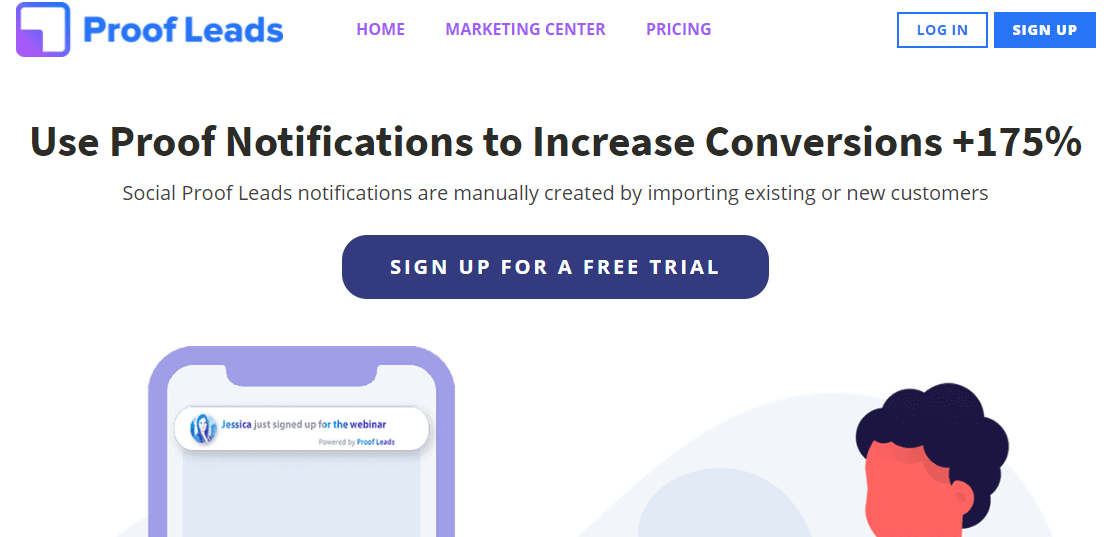The homepage of Proof Leads prominently features a clean and informative layout. In the top left corner, the Proof Leads logo is displayed in blue text, accompanied by a distinctive icon: a blue square with curved edges containing a smaller purple square inside. The navigation bar across the top in purple text offers links to Home, Marketing Center, and Pricing. On the right side of the navigation bar, there is a white button with a blue border labeled "Log In," next to a blue button with white text that reads "Sign Up."

Center stage on the page is a compelling headline in bold black font proclaiming, "Use Proof Notifications to Increase Conversions by 175%." Directly beneath this, a subtitle in thinner lettering explains, "Social Proof Leads Notifications are manually created by importing existing or new customers." A prominent navy blue button with white text invites users to "Sign Up for a Free Trial."

At the bottom of the page, a graphic illustration adds visual interest. On the left, an image of a phone displays a notification: "Jessica just signed up for the webinar powered by Proof Leads." To the right of this graphic, there is an illustration of a person with orange-coral skin and curly black hair, adding a human touch to the webpage.